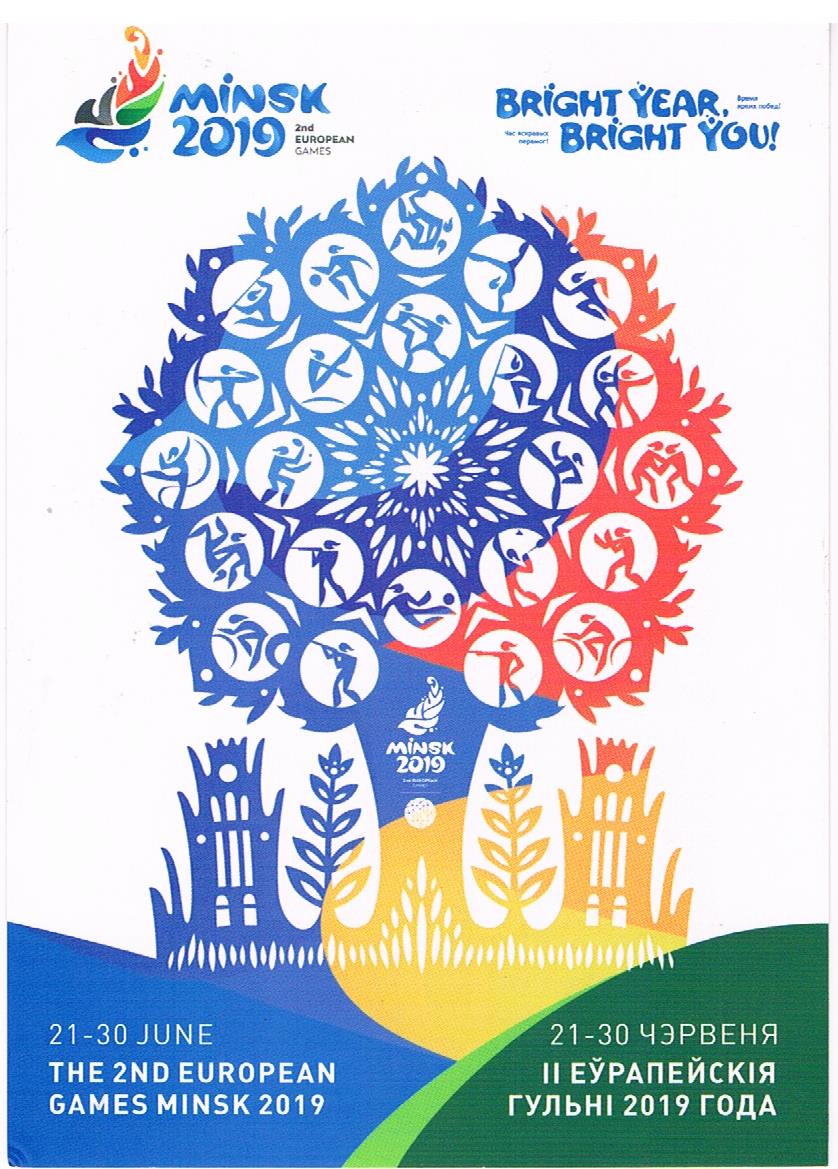This image is a detailed advertisement for the Minsk 2019 Second European Games. It appears to be a scan of a poster that might have been featured in a magazine. The poster's centerpiece is a large, colorful tree that emerges between two buildings. The tree is tinted in shades of blue and red, with various white circles embedded within its branches. Each circle depicts different sports and activities, including archery, canoeing, basketball, swimming, diving, wrestling, soccer, cycling, gymnastics, dancing, handstands, and more. The trunk of the tree prominently displays the text "Minsk 2019" along with a cornucopia-style symbol above it.

At the top of the image, written in bold blue text, is the phrase "Minsk 2019, Second European Games," accompanied by a rainbow-colored cornucopia symbol and the slogan "Bright Year, Bright You" in a watery blue text. The bottom of the advertisement specifies the event's dates, "21 to 30 June," and reiterates "the Second European Games Minsk 2019," also written in Russian. Small illustrations of castles and additional trees surround the bottom section, adding to the vibrant and dynamic design of the poster.